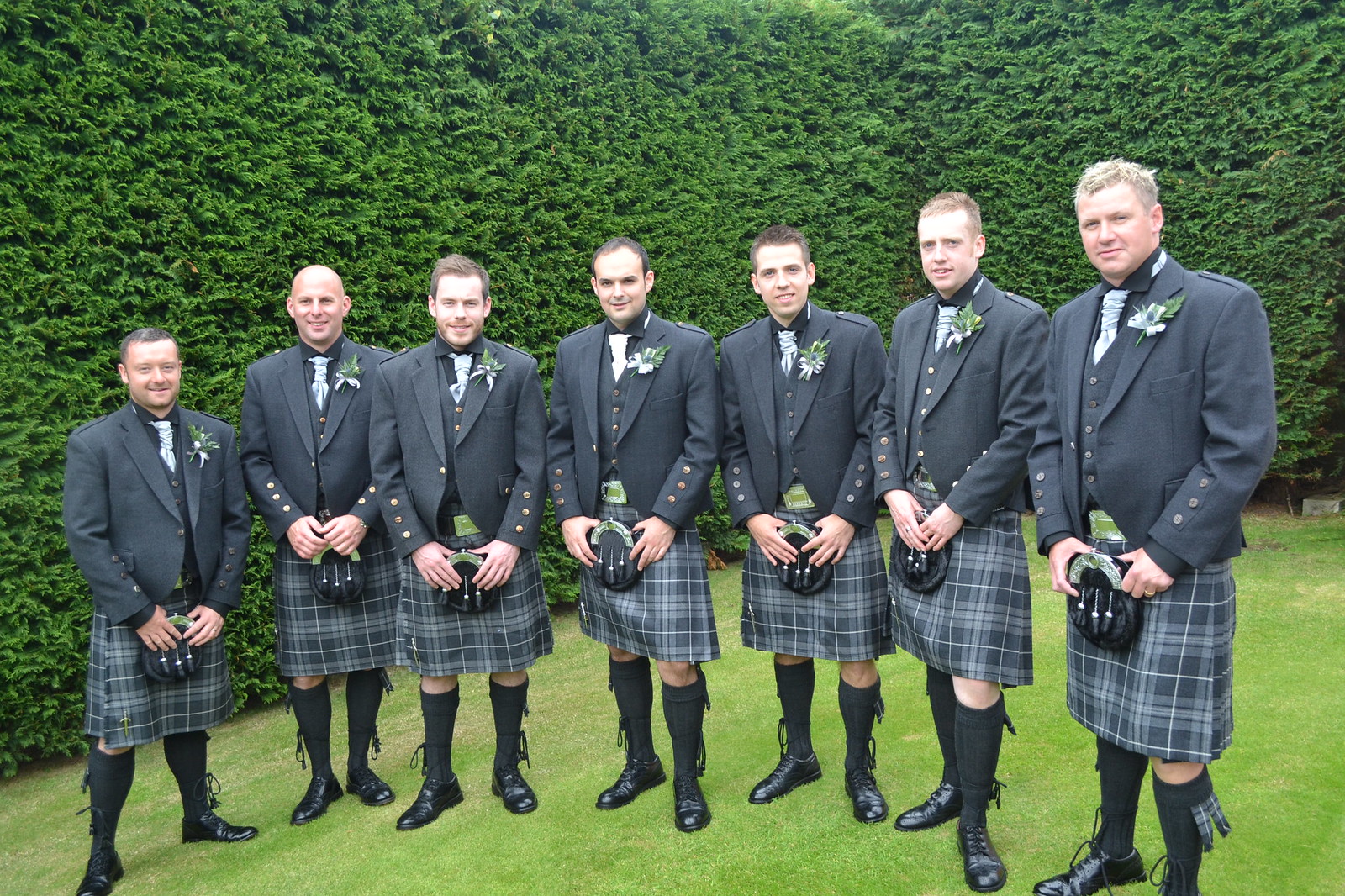In this photograph, seven Caucasian men are standing in a line on an impeccably manicured, bright green lawn reminiscent of a putting green. The background is framed by tall, uniform hedges. The men, appearing to be in their mid-20s to mid-30s, are dressed in matching ceremonial attire, likely for a significant occasion such as a wedding. They are wearing dark gray suit jackets, gray vests, gray shirts, and gray or white ties partially tucked into their vests. On their left lapels are white flowers with green leaves. Each man dons a dark and light gray checkered kilt reaching down to his knees, accompanied by gray knee-high socks trimmed with kilt material and black shiny dress shoes. Around their waists, they wear black leather sporrans with tassels and possibly silver tools. From left to right, the men vary in height and distinct features: short black hair, bald, brown hair with a mustache and short beard, black hair with a receding hairline, and blonde hair. They hold their hats or sporrans in front of their stomachs, and while some smile more than others, they all maintain a relaxed, confident demeanor as they look towards the camera.